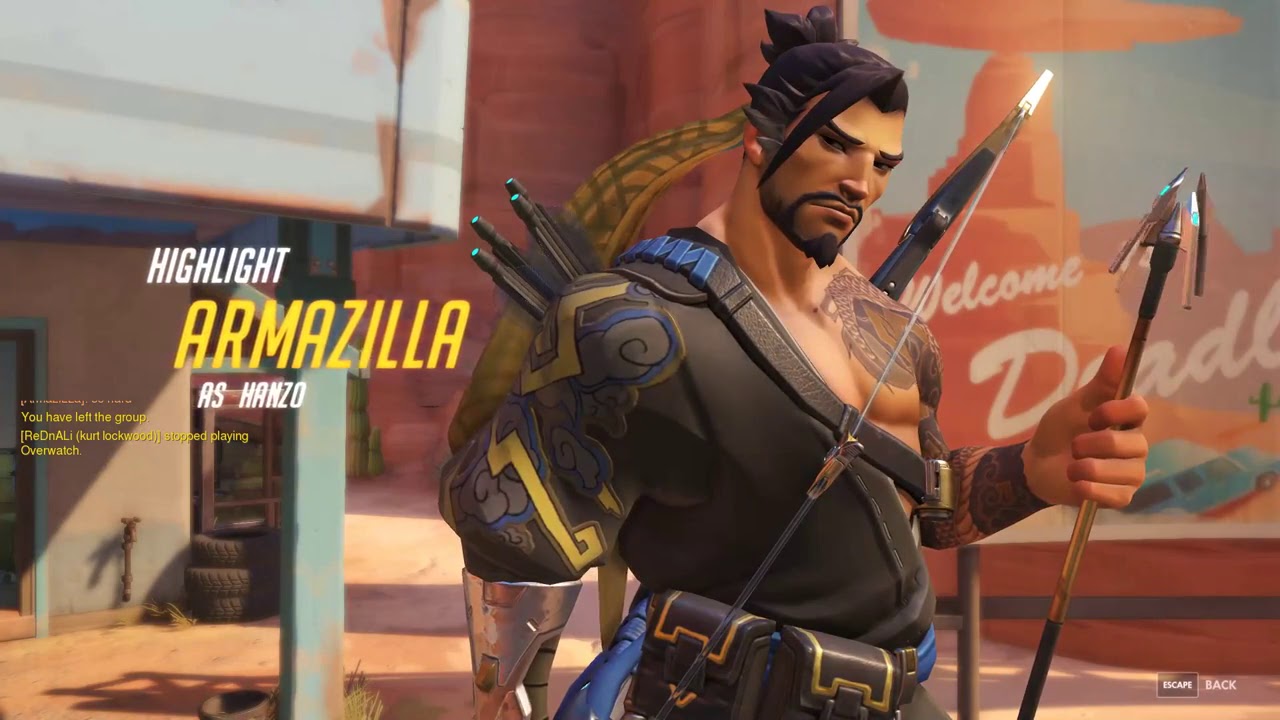The image depicts a detailed character select screen from a video game. The main character on display is identified as Armazilla, portrayed as Hanzo, as highlighted in capital white and yellow text on the left side of the screen. Hanzo is a 3D-rendered warrior garbed in a distinct half-shirt, resembling a black karate uniform adorned with gray line-drawn clouds and yellow lightning bolts on the sleeves. His right arm and shoulder are bare, revealing intricate tattoos extending to his chest. Hanzo's left arm is encased in a metallic wristguard and he clutches an arrow tipped with a silver point, with a bow draped across his chest and a quiver of arrows slung on his back. The character features black hair with a prominent strand falling to one side of his face, complemented by a black goatee and mustache.

The background shows an urban setting with a brick building and a green pillar supporting an entryway. Additionally, there's text that appears to read "Welcome Day Day," possibly a location in Florida. The lower right corner of the screen includes interactive buttons labeled "Escape" and "Back." A chat notification stating "You have left the group" is also present, adding to the immersive game environment. Overall, the image intricately blends character details with elements suggestive of dynamic gameplay.